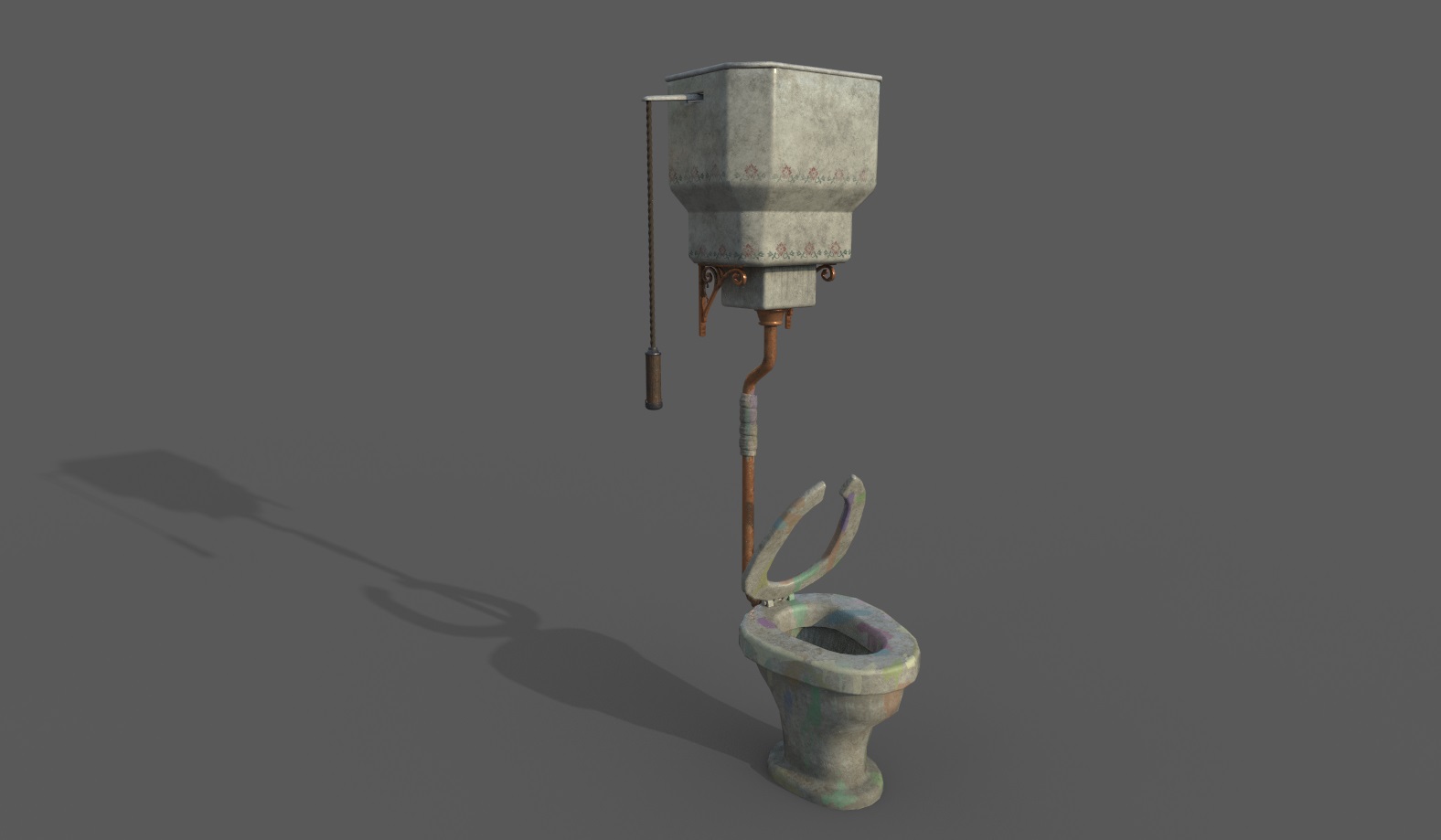The image showcases a 3D-generated model of a unique and somewhat surreal toilet set against a solid dark gray background. Central to the image, this toilet appears rusty and somewhat dirty, with a rainbow-colored base suggesting a mix of materials or age-related discoloration. The toilet bowl has its lid up, revealing what looks like steel construction with clear signs of rust.

A distinct feature of this model is its water tank, which is not positioned directly behind the toilet as usual but instead levitates above it, connected via a single copper-colored and slightly gray vertical pipe. This pipe extends upward to support a large, square-shaped tank that casts a shadow to the lower left, indicating light sourcing from the right side outside the image frame.

Another peculiar detail is the flushing mechanism. Unlike conventional designs, this toilet features a bar extending horizontally from the tank before dropping vertically halfway down its height to where it ends with a handle. This brownish bar and handle setup resembles a pull-string mechanism, adding to the toilet's unusual design.

Overall, the scene is void of any text, focusing solely on the CGI model of the toilet, its extended tank, and the shadow they cast on the gray floor.